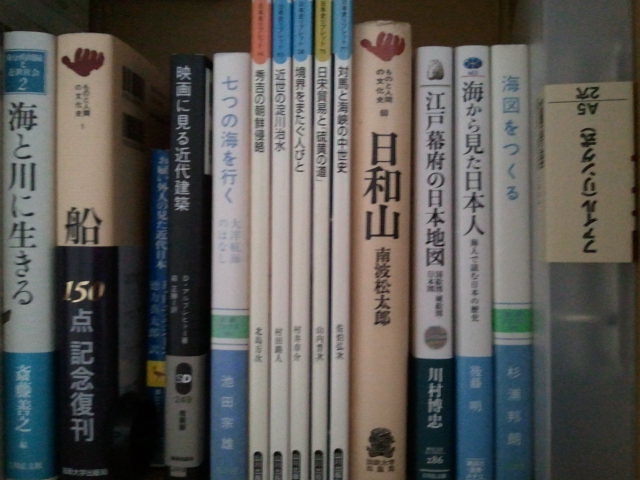The photograph captures a close-up view of the spines of various books neatly arranged on a brown wooden bookshelf. Each book displays Japanese writing on the spine, presented in a range of colors and styles. The collection includes both hardcover and paperback books of different widths. 

Distinctly in the center, there is a set of five tall, slender books, each with a colorful band at the top—red, two blues, green, and blue—while the rest of their covers are primarily white. Several of the books feature blue and white dust jackets, with a mix of blue, beige, and navy blue tones found throughout the lineup. Some specific details include a navy blue book with silver writing, a series of white books with blue bottoms, and a clear plastic binder with a beige label on the far right.

This visually organized bookshelf reflects meticulous care, with the arrangement showcasing both the books' aesthetic appeal and the owner's appreciation for Japanese literature.